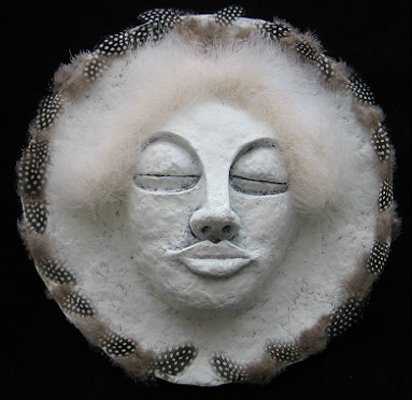The image features a circular sculptural object set against a completely black background. Dominating the center is a human-like face with closed eyes, characterized by a bold nose and prominent lips, giving it a primitive, almost ancient appearance. Surrounding the face, the circular frame is adorned with intricate black and white polka-dotted patterns and what appear to be black and white feathers or hair-like features, creating a halo effect. The face itself is sculpted from a material that could be white clay or rock, suggesting it is handmade and possibly crafted by an indigenous artist. The object, which evokes a sense of being a mask or relic, exudes a strong artistic and museum-worthy presence, featuring shades of black, white, tan, and gray. The entire sculpture takes up most of the image, with only the corners revealing the dark background, emphasizing its central and captivating position.